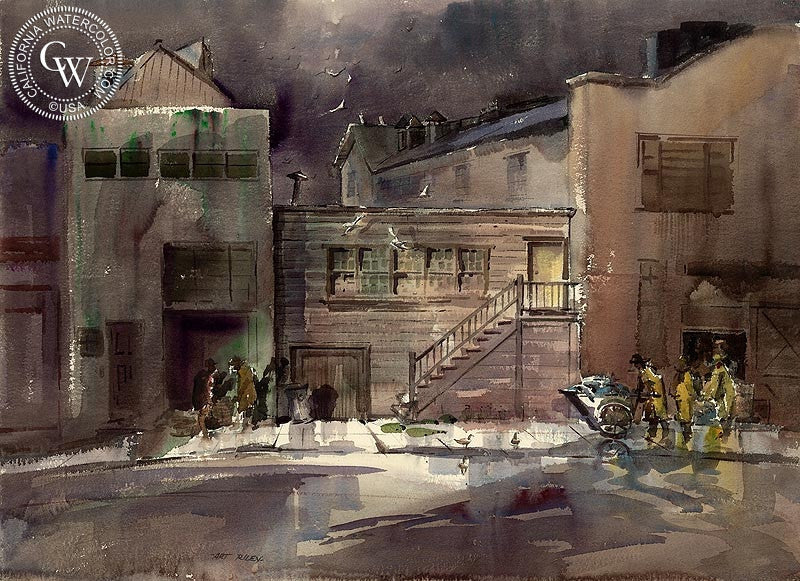The image is a detailed, vintage-style watercolor painting, predominantly featuring dark hues of browns, blacks, and grays, accentuated with reflections that suggest a wet cement ground with intermittent puddles. It depicts an old cityscape with multiple buildings, each two to three stories high, constructed of stone. One notable building on the left side has five windows across its top. There’s another building on the right side with stairs leading up to it, near which are people wearing indistinguishable yellow or gold outfits. These figures are pushing wheelbarrows filled with assorted items and are painted in a manner that lacks fine detail. The background features a dark, stormy sky blending black and gray colors. Above the scene, there is a circular logo that reads "California Watercolor.com" along with "CUSA," and has "CW" prominently featured in the center. The entire composition has an abstract, heavy watercolor appearance with a focus on the moist street and intricate old architecture.